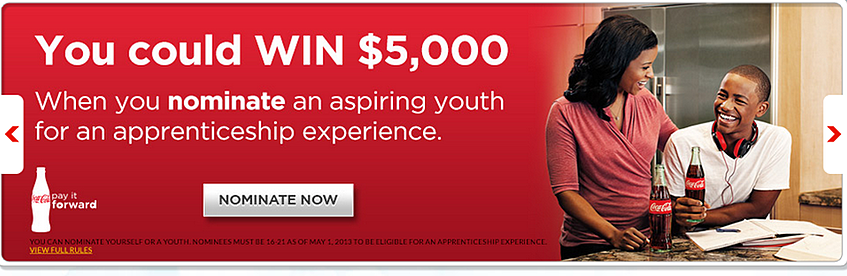Banner Ad Description:

The Coca-Cola Company has created a visually engaging banner ad for their "Pay It Forward" campaign, hosted on their website. Dominated by Coca-Cola's signature red and white colors, the ad features an inspiring image of an African-American mother engaging warmly with her son, who appears to be an enthusiastic, aspiring youth working on homework in their cozy kitchen setting.

Above the image, bold text announces the opportunity to "Win $5,000" and calls for nominations of promising young individuals for a valuable apprenticeship experience with Coca-Cola. A prominent, large white button in the center of the banner invites visitors to "Nominate Now."

The iconic Coca-Cola bottle is also showcased, enhancing brand recognition and reinforcing the ad's connection to the company's esteemed reputation. Viewers are encouraged to nominate deserving young African-American candidates, giving them a chance to gain invaluable experience while also potentially rewarding the nominator with a significant monetary prize.